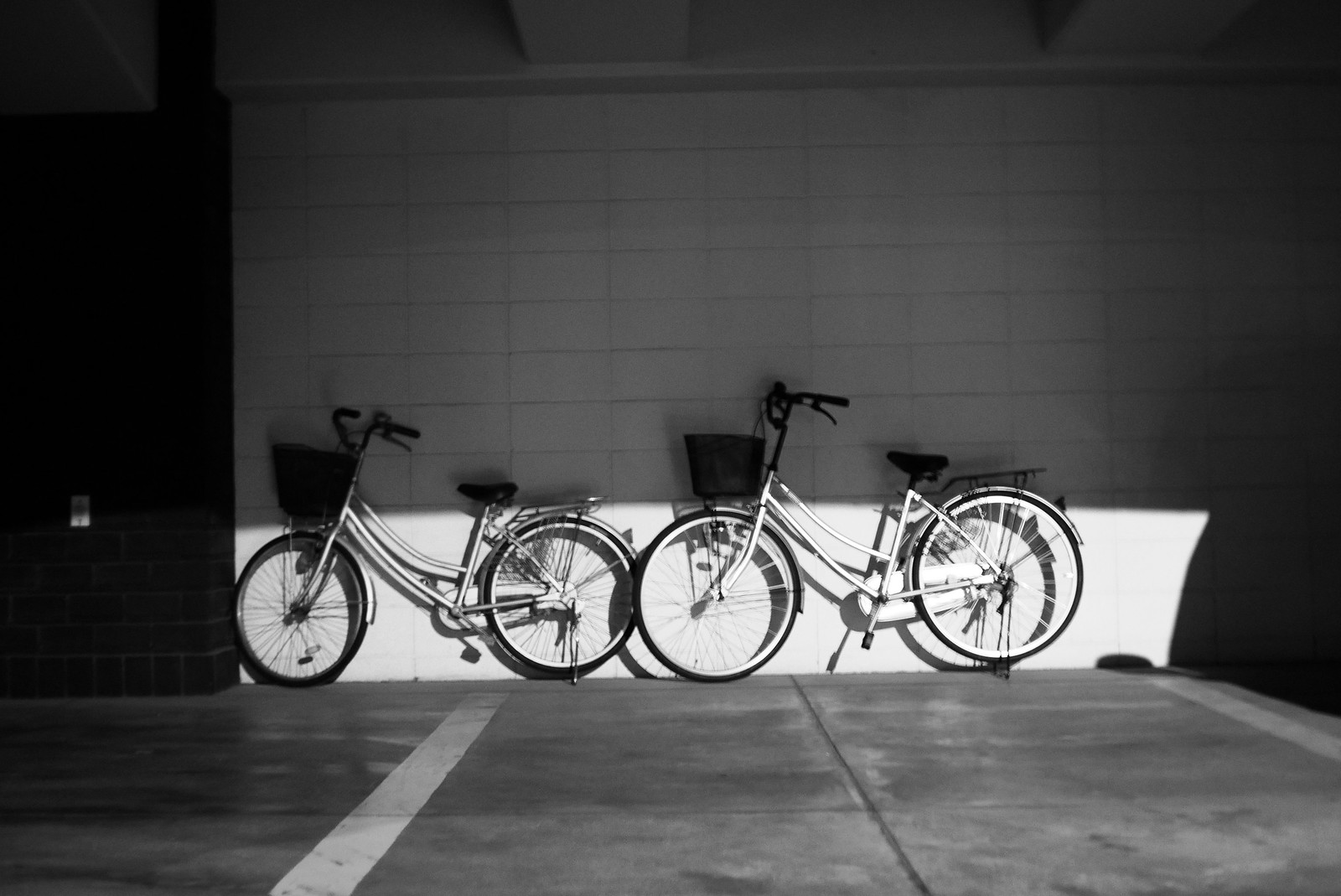This black and white photograph captures a pair of adult-sized bicycles parked side by side against a white brick wall in what appears to be a parking lot. The bicycles, which are facing left, feature white frames, black seats, and black baskets attached to their handlebars. They also have white-rimmed tires that stand out distinctly. The scene includes a gray concrete floor marked with white stripes, adding to the structured environment. The left bicycle touches a black brick wall that contrasts with the otherwise predominantly light-colored setting. Sunlight illuminates the lower parts of the bicycles, highlighting their wheels and body, while shadows cast by an overhead structure obscure the upper parts and wall behind them. This artistic composition blends stark contrasts and subtle textures, providing a visually compelling image.